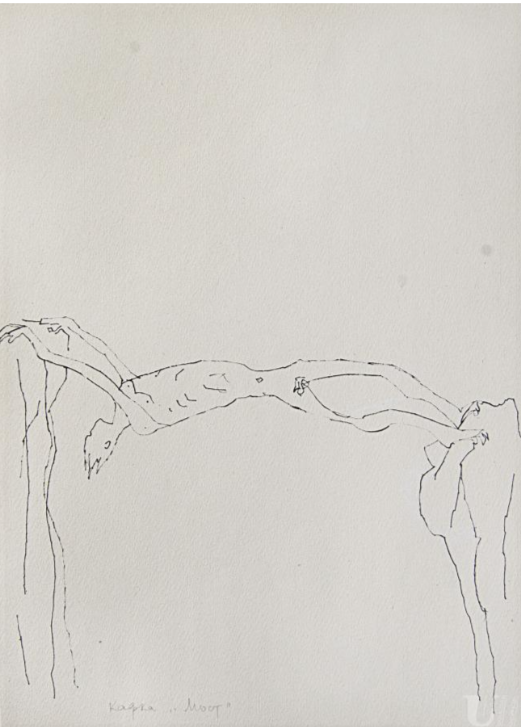This image is a simplistic yet emotional line drawing on plain white paper. It depicts a malnourished, unclothed human figure stretched horizontally between two vertical stone cliffs or posts. The background is predominantly white with minimal details. The figure's upper arms are gripping onto the left post, while their long, skinny legs are curled around the edge of the right post for support. The individual's posture suggests they are hanging precariously with their stomachs facing upward and their heads dangling downwards, accentuating their ribcage and navel. Additionally, a small leaf covers the lower midsection of the body. Notably, the composition is signed at the bottom center with a barely legible signature possibly beginning with a 'K' or 'N'. Despite its simplicity, the drawing conveys a strong sense of struggle and fragility.